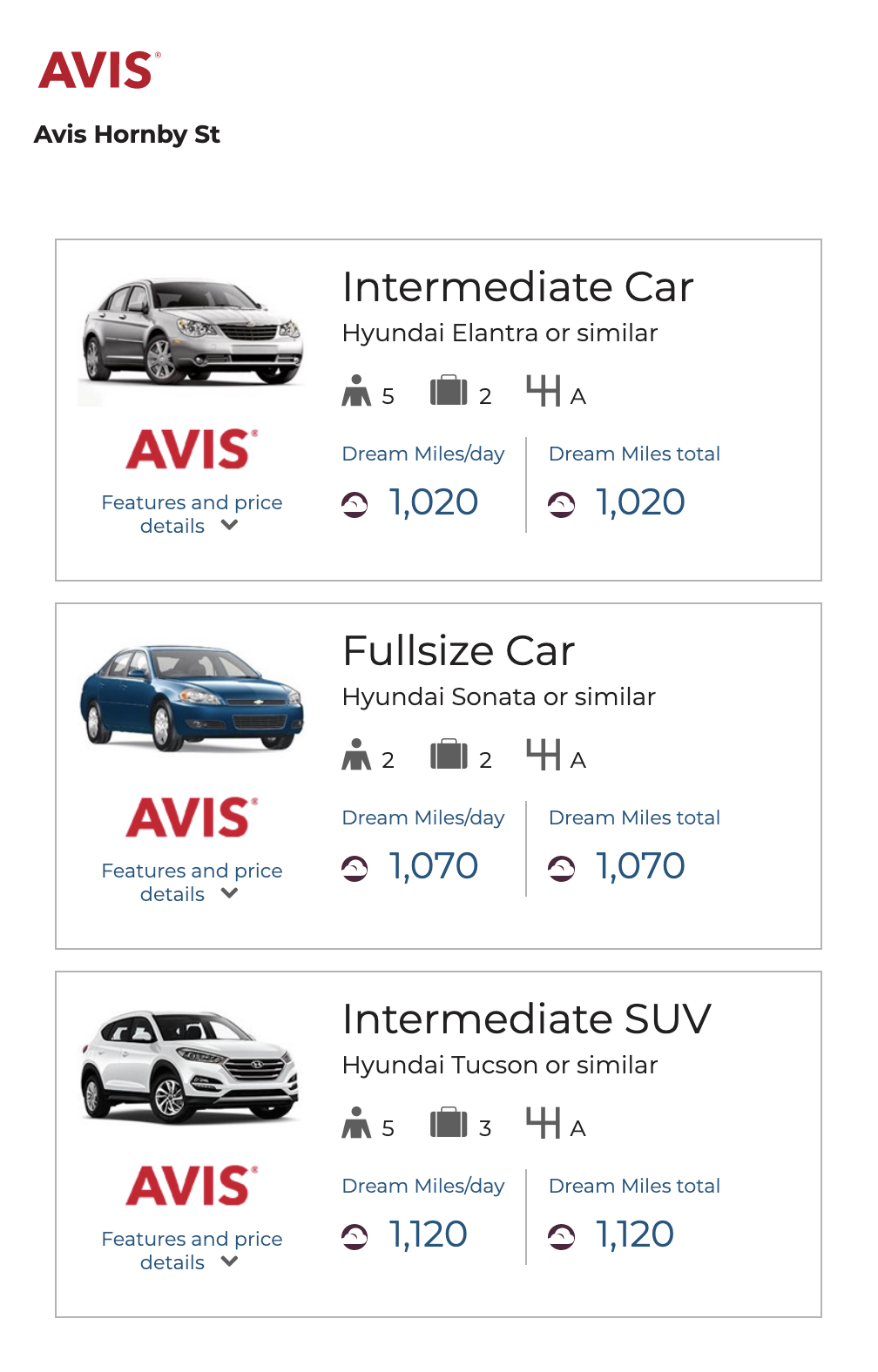The image appears to be a screenshot from a mobile phone, showcasing a car rental listing from Avis. The interface is displayed on a clean white background in a vertical rectangular format.

At the top left corner, there's the red Avis logo followed by "Avis Hornby ST" written in black. Below this heading, there are three distinct rectangular boxes detailing available car rental options:

1. **Intermediate Car: Hyundai Elantra or Similar**
   - A graphic of a silver car with a red Avis logo underneath.
   - **Seats:** 5 people
   - **Luggage:** 2 suitcases
   - **Dream Miles per Day:** 1,020
   - **Dream Miles Total:** 1,020
   - A blue link labeled "Features and Price Details" is provided for more information.

2. **Full-Size Car: Hyundai Sonata or Similar**
   - A graphic of a blue car with a red Avis logo underneath.
   - **Seats:** 2 people
   - **Luggage:** 2 suitcases
   - **Dream Miles per Day:** 1,070
   - **Dream Miles Total:** 1,070
   - A blue link labeled "Features and Price Details" is provided for more information.

3. **Intermediate SUV: Hyundai Tucson or Similar**
   - A graphic of a silver SUV with a red Avis logo underneath.
   - **Seats:** 5 people
   - **Luggage:** 3 suitcases
   - **Dream Miles per Day:** 1,120
   - **Dream Miles Total:** 1,120
   - A blue link labeled "Features and Price Details" is provided for more information.